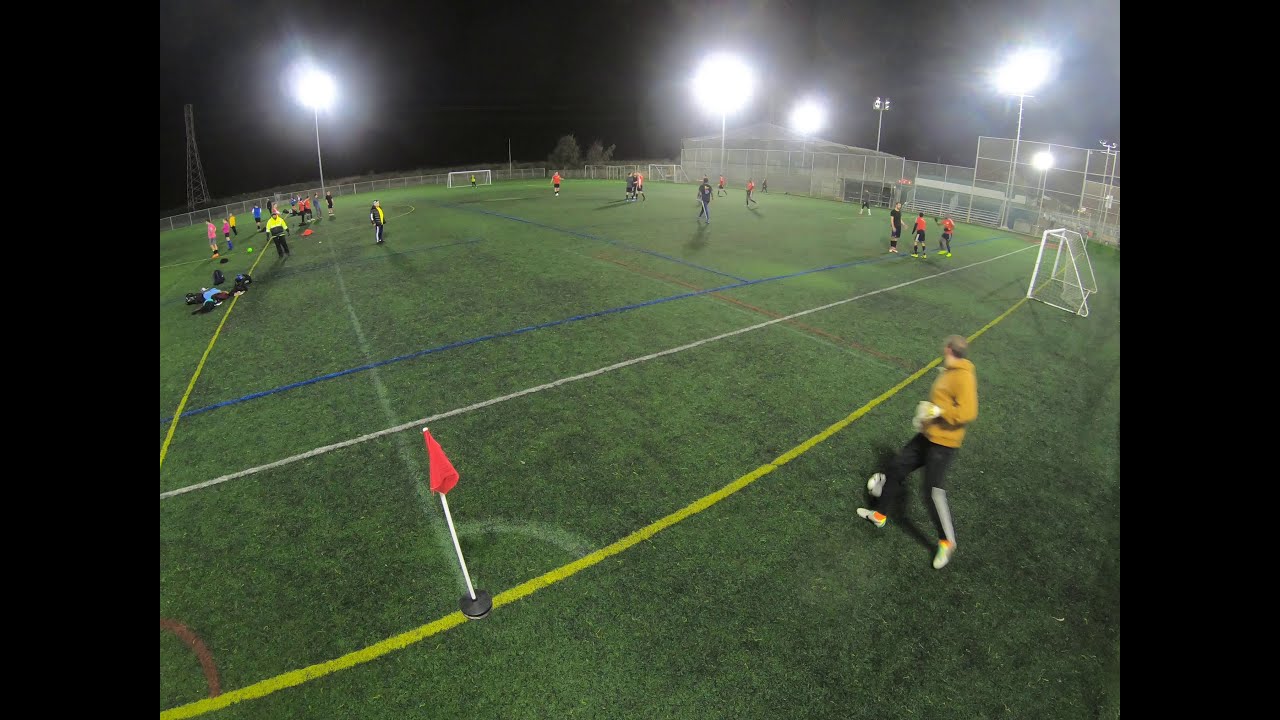The image captures a nighttime scene on a well-lit soccer field with several bright stadium lights illuminating the dark sky. The field is lush and green, marked with yellow, blue, and white lines, indicating various boundaries and sections. On the left side of the field, there is a prominent red flag marking the sideline. A man dressed in a yellow hoodie and black athletic pants is poised to kick a white soccer ball that rests near his right foot. The scene suggests there might be two games or practice sessions happening simultaneously, as there are large groups of players in various colored jerseys—red and yellow—dotting both sides of the field. In the background, two goals are visible, and to the far right, there's a fenced area likely used for other sports like tennis or badminton. Although there are bleachers set up, they appear to be empty, hinting that this might be a practice session rather than an actual game.